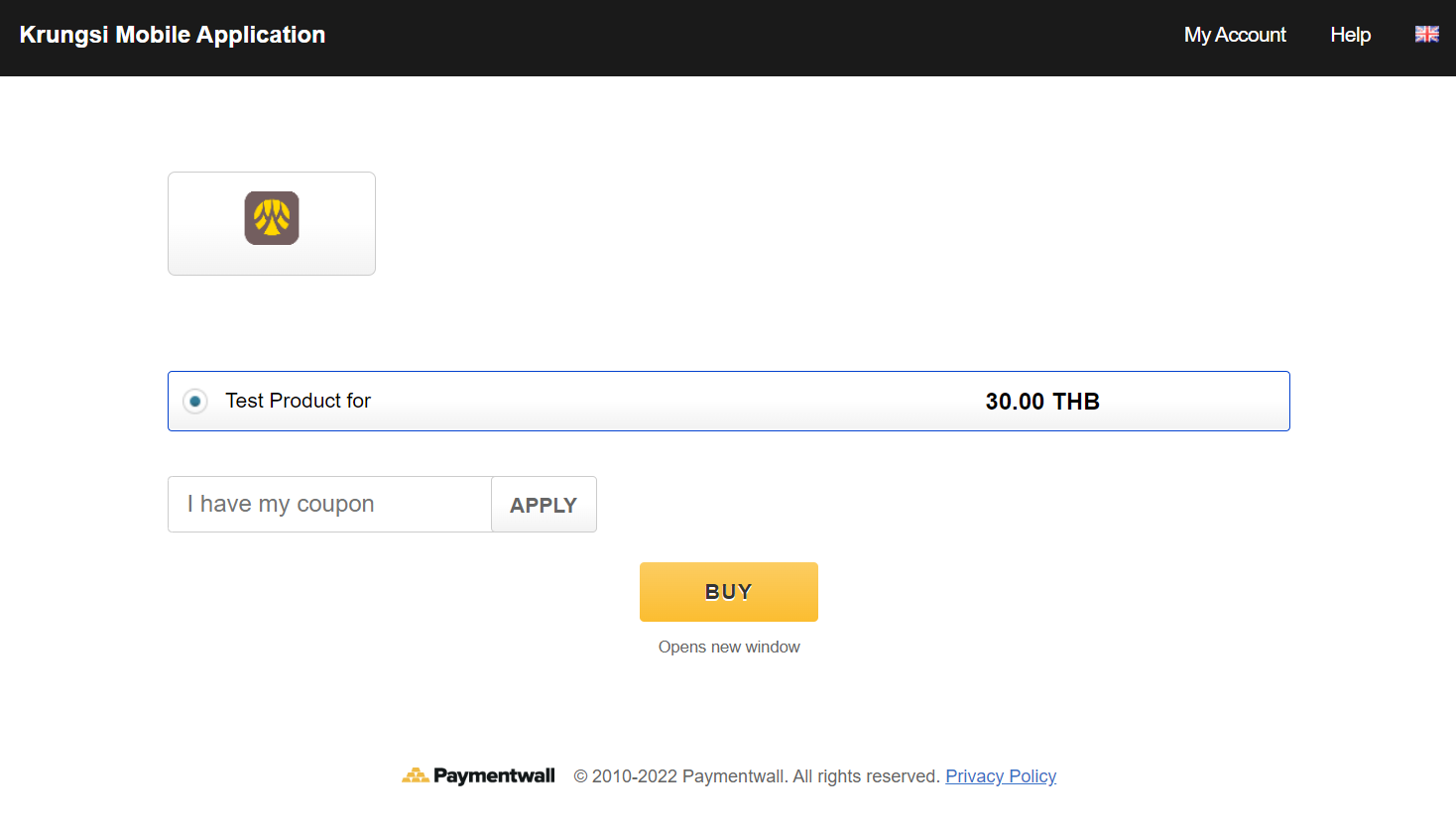The image depicts a computer screen primarily displaying a white background. At the top, a thin horizontally placed dark band runs across the screen. On the left side of this band, the text "Krungsi Mobile Application" is displayed in white letters. Notably, "Krungsi" is spelled with a capital 'K' followed by "R-U-N-G-S-I." To the right of this band, also in white, are the options "My Account" and "Help," with a British flag displayed at the far right end.

Below this dark band, the screen returns to a white background where a gray-outlined rectangle is centered. This rectangle, though mostly white, has a distinct design in the middle featuring a brown square with a yellow circle within it, potentially depicting mountains drawn in brown.

Further down, a horizontal selection bar appears with a blue-highlighted option button labeled "Test Product 4." To the right of this option, the price is displayed as "30.00 THB."

Below the product selection, there is a text response box with the phrase "I have my coupon" typed in. Adjacent to this response box is a clickable "Apply" button.

Centered on the screen just below the response box, there is a gold-colored button with the word "Buy" in black text. In small, dark letters under this button, it reads "Opens New Window."

At the very bottom of the screen, there is a small, centered triangle composed of nine gold dots. To the right of this triangle, the words "Payment Wall" are printed in dark letters. Below this, in smaller, lighter text, it reads "Copyright 2010 to 2022 Payment Wall. All Rights Reserved. Privacy Policy." The phrase "Privacy Policy" is underlined and in blue, indicating it is a clickable link.